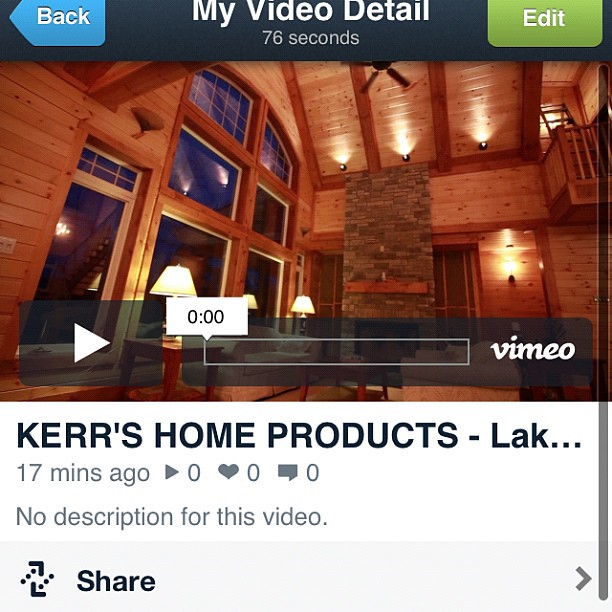This is a detailed photograph of a computer screen displaying a Vimeo video inside a white-themed application or website. The focus is on a video titled "KERS Home Products / Lake," which captures the interior of a wooden house. The house's room features high wooden walls, a ceiling fan, skylights, a brick fireplace that extends to the ceiling, and large windows. Above the video is a blue bar that reads "My Video Detail, 76 seconds." On the left side of this bar is a blue "Back" button, and on the right side is a green "Edit" button. Just below the video, it notes "17 minutes ago," accompanied by "zero arrows, zero likes, zero comments." The description states there is no description provided for the video.